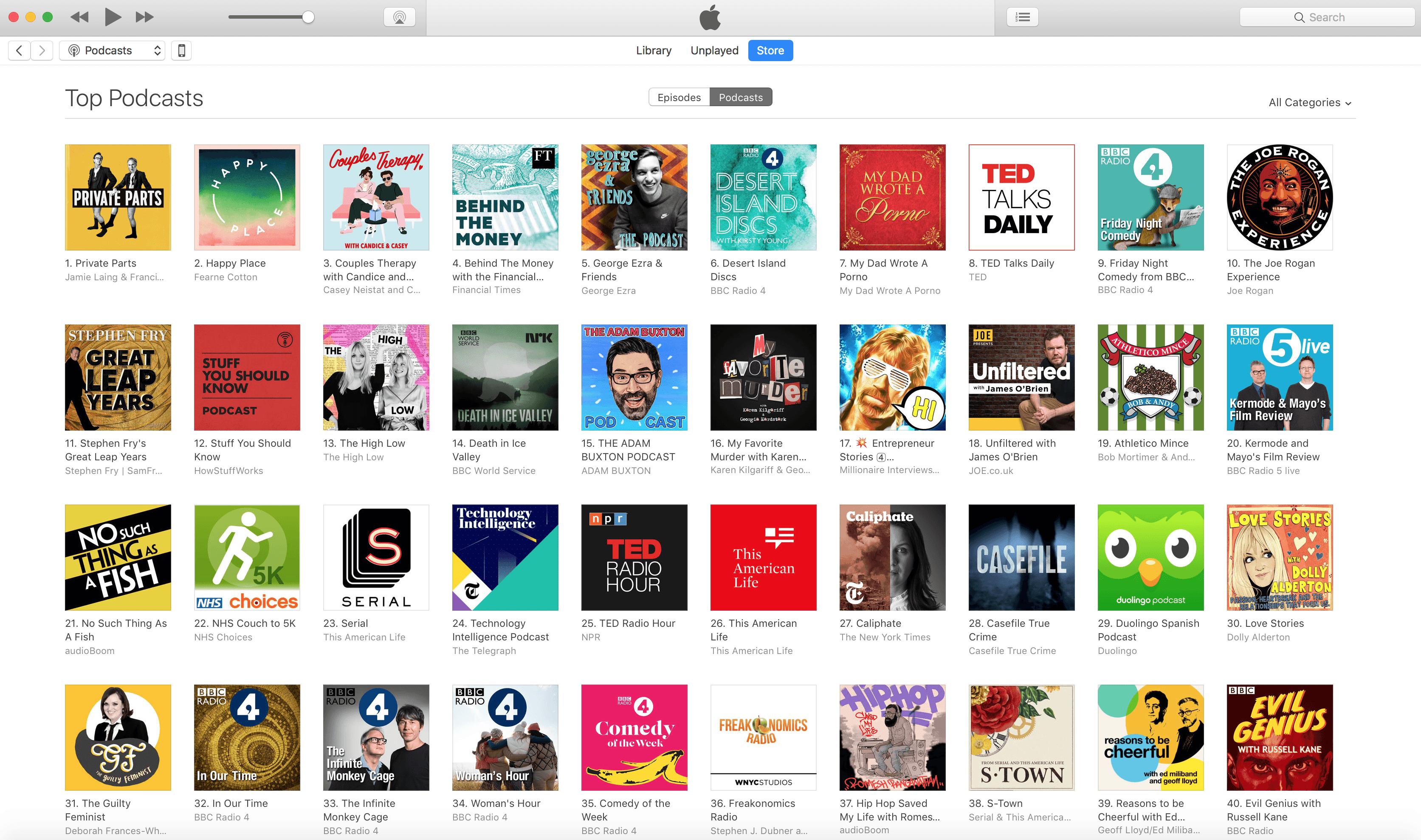A detailed caption for the provided image could be:

The image displays a personalized podcast library page from an Apple device. The interface is clean and structured, featuring the characteristic yellow, red, and green dots in the upper left corner consistent with the macOS window design. Across the top, there are options for 'Library,' 'Unplayed,' and 'Store.' Below these tabs, two categories 'Episodes' and 'Podcasts' are available for navigation, supplemented by a search option and a context menu on the right side. A highlighted dropdown menu indicates that the user is currently viewing podcasts from 'All Categories.'

The central section of the page lists various podcast titles that the user follows, from top to bottom, in the following order: 
- Private Parts
- Great Leap Years
- No Such Thing as a Fish
- The Guilty Feminist
- Happy Place
- Stuff You Should Know
- The 5K Choices
- In Our Time
- Coyote Therapy
- Couples Therapy
- The High-Low
- Serial
- The Infinite Monkey Cage
- Behind the Money
- The Death in Ice
- Technology, Internet Podcast
- Women's Hour
- The George Ezra and Friends
- The Adam Buxton Podcast
- TED Radio Hour
- Comedy of the Week
- Desert Island Discs
- Favorite Murder
- American Life
- Freakonomics Radio
- My Dad Wrote a Porno
- Entrepreneur Stories
- Celeb at Home
- S-Town
- Friday Night Comedy
- American Minutes
- Duolingo Spanish Podcast
- Reasons to be Cheerful with Ed
- The Joe Rogan Experience
- Kermode and Mayo's Film Review
- Love Stories
- The Evil Genius with Russell Kane

These podcasts represent a diverse array of genres and interests, indicating a wide variety of content available for the user to enjoy on their Apple device.